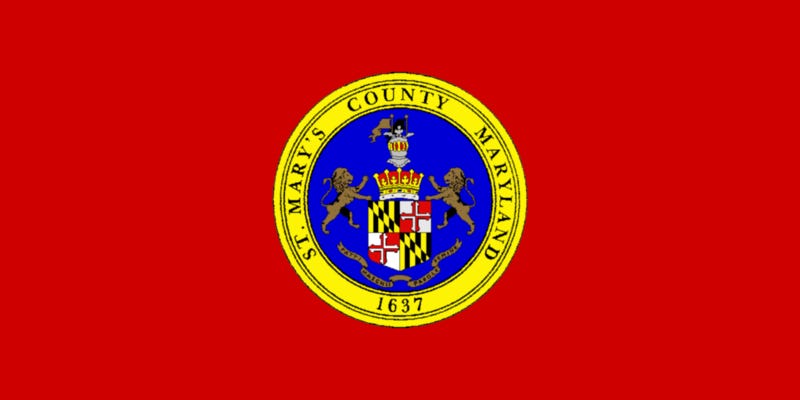The image depicts a horizontal rectangular flag with a red background. Centered on the flag is a yellow circle with a blue interior. Encircling the blue field, in black text, are the words "St. Mary’s County, Maryland, 1637," indicating the county's establishment year. Inside the blue circle lies a detailed coat of arms. At the top of the crest rests a medieval knight's helmet adorned with a crown, and above the helmet is a trophy-like figure with flags. The shield beneath the crown is divided into four sections: a yellow and black geometric pattern, and red and white areas featuring arrows and a cross. Flanking the shield are two lions poised on their hind legs, and beneath the shield is an unreadable banner.